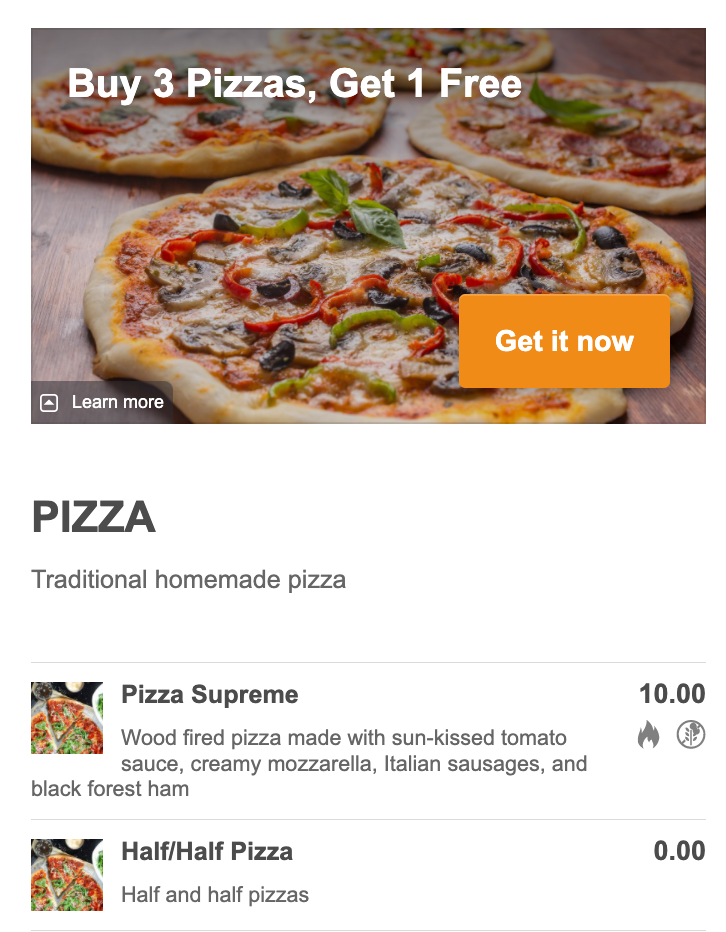This vibrant promotional image showcases an enticing "Buy Three Pizzas, Get One Free" offer. Central to the composition are four distinct pizzas, each laden with an array of fresh, colorful toppings, hinting at the variety available. The story starts at the top with an image featuring a pizza and a "Get It Now" call-to-action button prominently positioned at the bottom right, enticing viewers to take immediate advantage of the offer. At the bottom left of this section, another button labeled "Learn More" invites further exploration.

The detailed descriptions of the pizzas reveal their mouth-watering appeal: 

1. **Traditional Homemade Pizza** - A classic favorite, topped with sun-kissed tomato sauce, creamy mozzarella, Italian sausages, and Black Forest ham.
2. **Pizza Supreme** 
3. **Wood-Fired Pizza** - Made with sun-kissed tomato sauce, creamy mozzarella, Italian sausages, and Black Forest ham.
4. **Half-Half Pizza** - A combo option featuring two flavors.

The color palette of the image is both vibrant and appetizing, with dominating hues of red, green, brown, orange, and black set against a predominantly white background, which highlights and amplifies the vividness of the pizzas. This visual contrast makes the image pop, drawing the viewer's eye to the delicious offerings and the compelling deal.